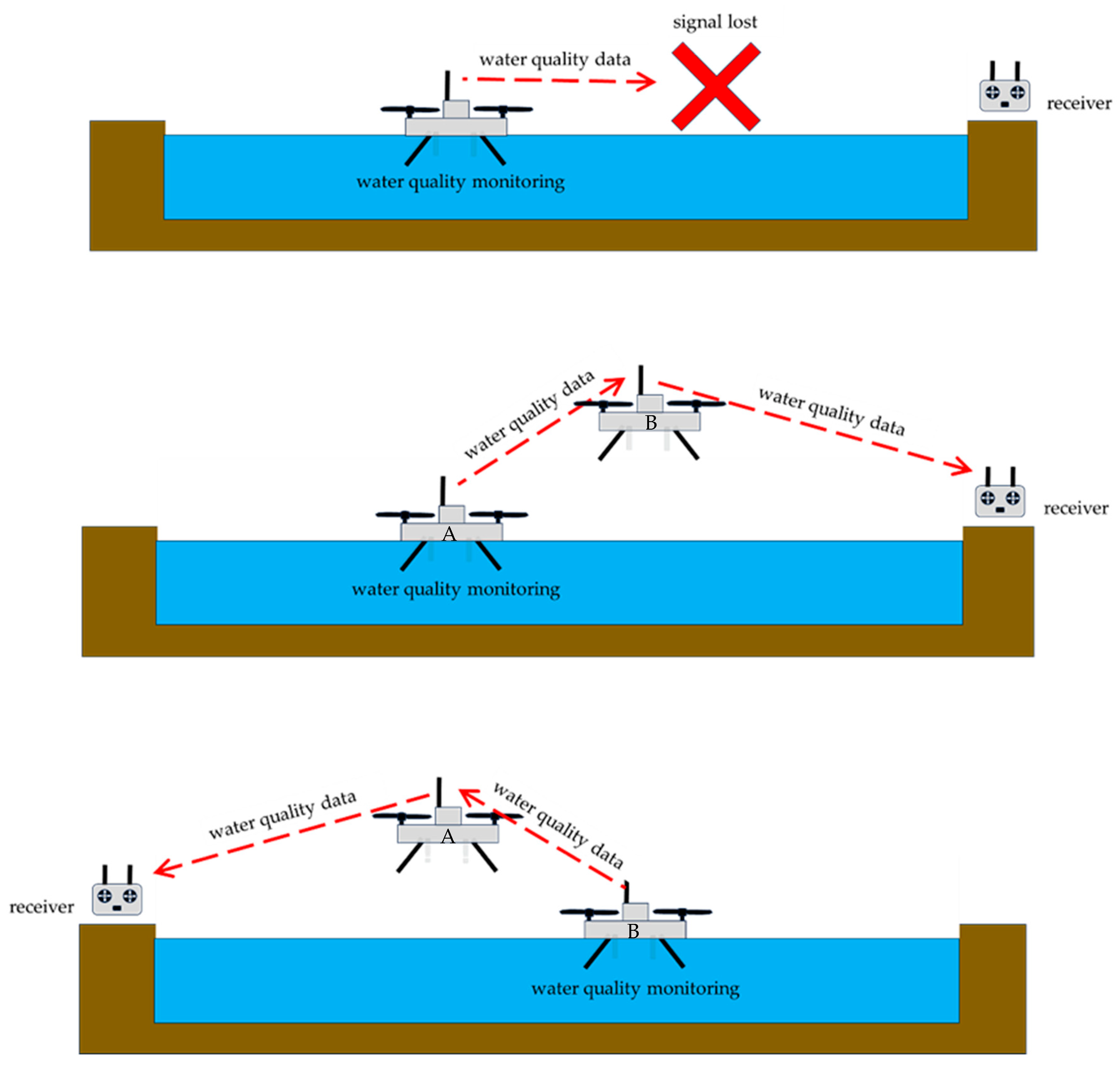The image is a simple, hand-drawn or computer-generated diagram illustrating a water quality monitoring device and its interaction with a receiver. The diagram is split into three sections, each depicting different scenarios of signal transmission. 

In all sections, the illustration features a brown pool representing the body of water, filled with blue water color. Inside the pool, there's a gray, mechanical-looking water quality monitoring device that is responsible for measuring water quality data. 

In the first section at the top, the receiver is positioned on the right, and the monitoring device is on the left within the water. A red, dotted line labeled "water quality data" extends from the device to an 'X' mark, indicating that the signal is lost.

The second section beneath it shows the monitoring device and receiver on the same side of the pool. Here, the red, dotted line, also marked "water quality data," successfully transmits from the monitoring device to the receiver, demonstrating successful signal transmission.

In the bottom section, the setup flips again, with the receiver on the left and the water quality monitoring device on the right. A secondary transmitting device is now placed on the left side, enabling the signal, depicted by the red, dotted line labeled "water quality data," to be effectively relayed to the receiver. 

Text annotations clarify the device positions and the success or failure of signal transmission labeled as position A and position B. Overall, the diagram provides step-by-step instructions on how to properly position the water quality monitoring device to ensure accurate data transfer to the receiver.